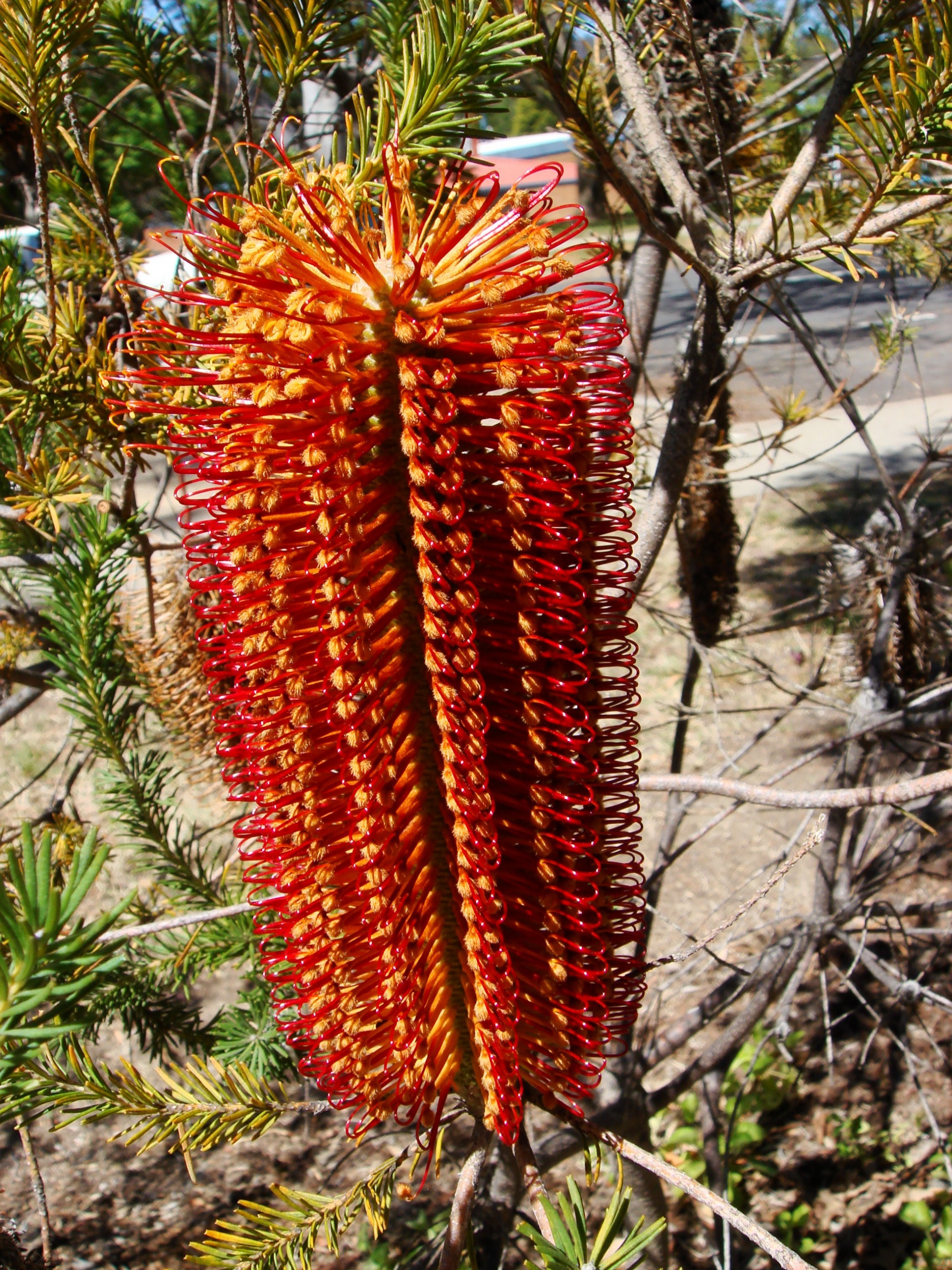The image captures a vertical rectangular scene of an unusual and vibrant plant, showcasing a striking flower or cone structure protruding from a tree or bush. The plant features a cylindrical shape with prominent sections segmented into several columns. These columns are adorned with numerous needle-like or loop-shaped projections in a very vibrant red color, transitioning to a yellow or orange hue towards the center. The entire structure, estimated to be about 18 to 24 inches tall and 12 inches wide, appears sticky or has flowering elements on it, adding to its unique texture.

In the foreground, tree branches with pine needles can be seen surrounding the plant. The background includes a street with white dashed lanes and a mailbox visible, set against a backdrop of additional trees and ground plants. The scene is bathed in natural outdoor light, with the ground itself being brown, indicative of an earthy setting. The image provides a detailed look at this fascinating botanical specimen that is both unusual and visually captivating.